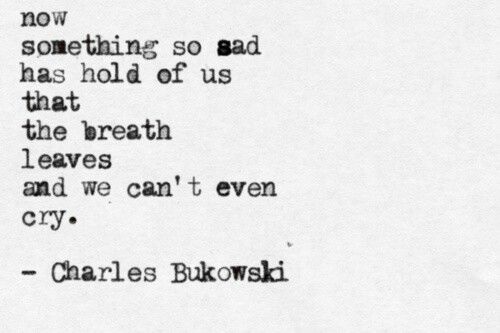This is a photograph of an off-white, light gray rectangular piece of paper featuring a poem by Charles Bukowski, typed in black ink with imperfect, analog typewriter-like font. The text is entirely lowercase, left-aligned, and comprises eight short lines, each subsequent line building upon the previous one: "now something so sad has hold of us that the breath leaves and we can't even cry." The typeface exhibits inconsistencies with some characters appearing smudged and others darker or lighter, contributing to its raw, imperfect appearance. Near the bottom, below the poem, "Charles Bukowski" is typed with proper uppercase and lowercase letters. The right side of the paper is largely blank, and there is slightly more space below the poem than above it.